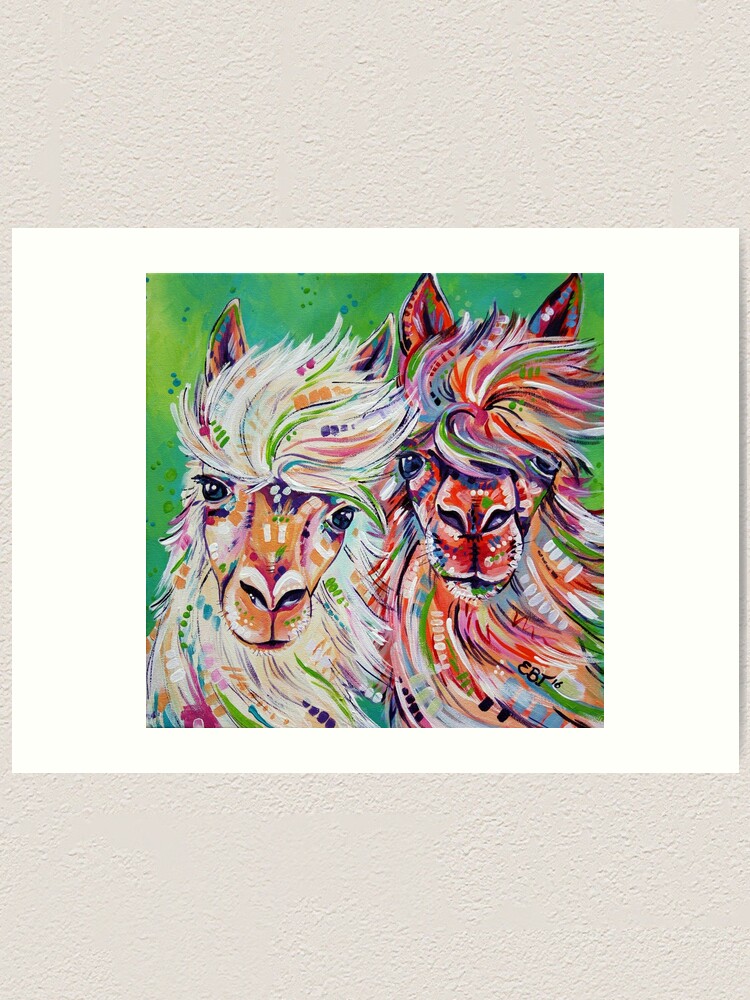The image depicts a captivating piece of digital artwork set against a vertically oriented, beige plastered wall. Centrally positioned within the composition, a rectangular white canvas showcases a vivid portrayal of two llamas. The background of the artwork is a lively green adorned with sporadic bluish-green dots. The llama on the left features predominantly white fur interspersed with splashes of orange, green dots, and wisps of blue, pink, and green. Its snout is mainly orange, and its ears flaunt a mix of varied hues. Contrastingly, the llama on the right is even more vibrant, with its fur richly imbued with red and pink shades, complemented by multicolored patches, especially noticeable on its snout, hair, and ears. Both llamas exhibit a fur texture that is whimsically wispy and multi-hued, imparting a sense of movement and depth. The detailed craftsmanship is further enhanced by the clean white borders surrounding the painting, which provides a crisp frame to the overall imagery. Additionally, the bottom right corner of the artwork contains a signature in black writing, appearing to read "EBT," attributing the piece to the artist.